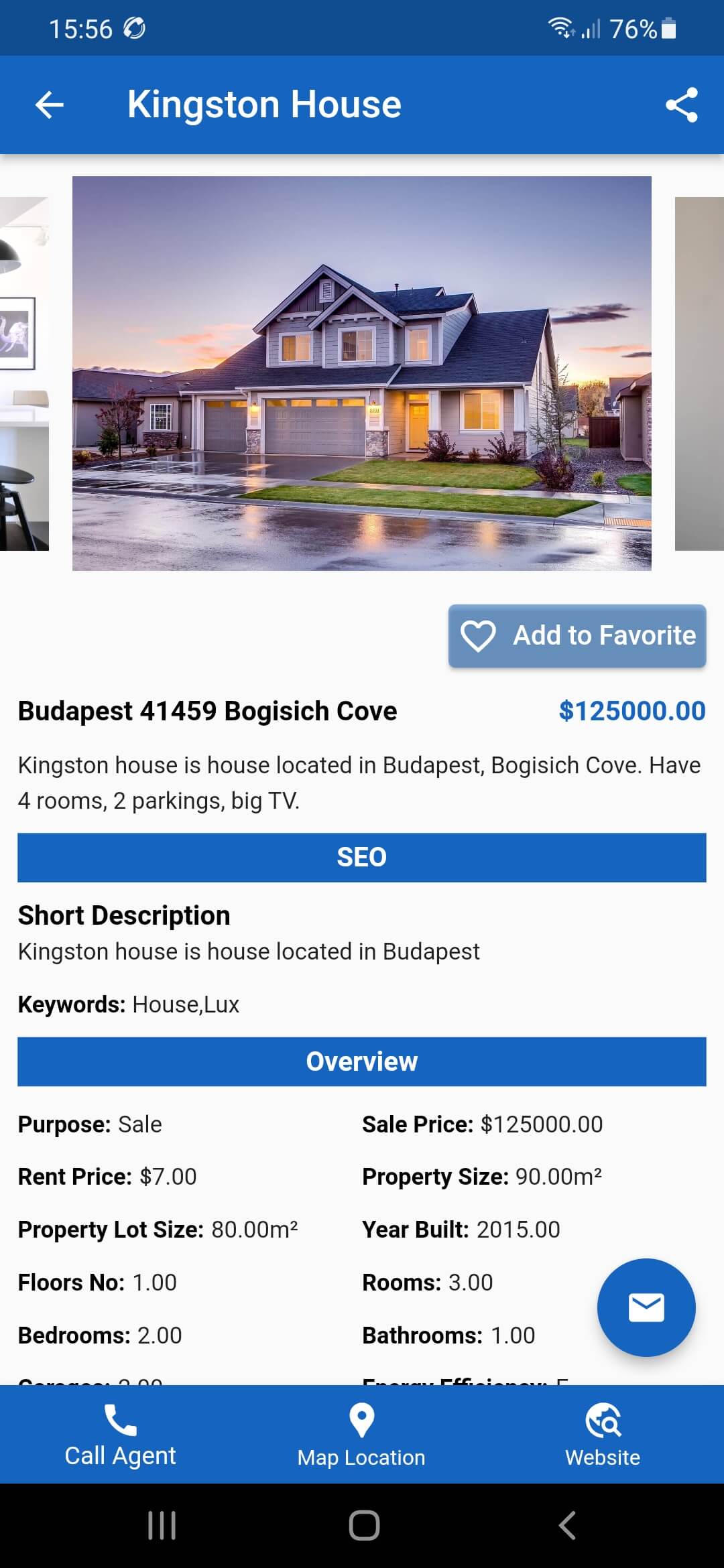This vertically oriented image, captured from a smartphone device, features a detailed display of a real estate listing for a home called Kingston House, located in Budapest. At the top of the screen, set against a navy or dark teal background, the status bar shows the time as 15:56 in military format, along with a notification icon. On the right side of the status bar, Wi-Fi, signal strength bars, and a 76% battery life icon are visible. Below the status bar, a white arrow pointing left is seen next to the text "Kingston House," accompanied by an additional white icon on the right.

Directly below this, an image of the property is displayed, showcasing the home’s exterior including the road, driveway, and a small grassy area. The two-story house is prominently featured in the picture. An interactive button labeled "Add to Favorite" is located within this section, alongside the address and listing price of 125,000. 

Further information reveals that Kingston House, positioned on Bacasevic Cove, includes four rooms, two parking spaces, and a large TV. A white box labeled "SEO" contains a brief description: "The Kingston House is a house located in Budapest," and mentions keywords related to the house's appearance.

Additional details are provided in a blue box titled "Overview," which specifies that the property is available for sale at 125,000. The lot size is 80 square meters with a build size of 90 square meters, featuring two floors, three rooms, one bedroom, and one bathroom, constructed in 2015. 

At the bottom, options for contacting an agent, viewing a map location, and accessing a website are available. The screen's footer consists of a black rectangle with three clickable icons for further navigation.